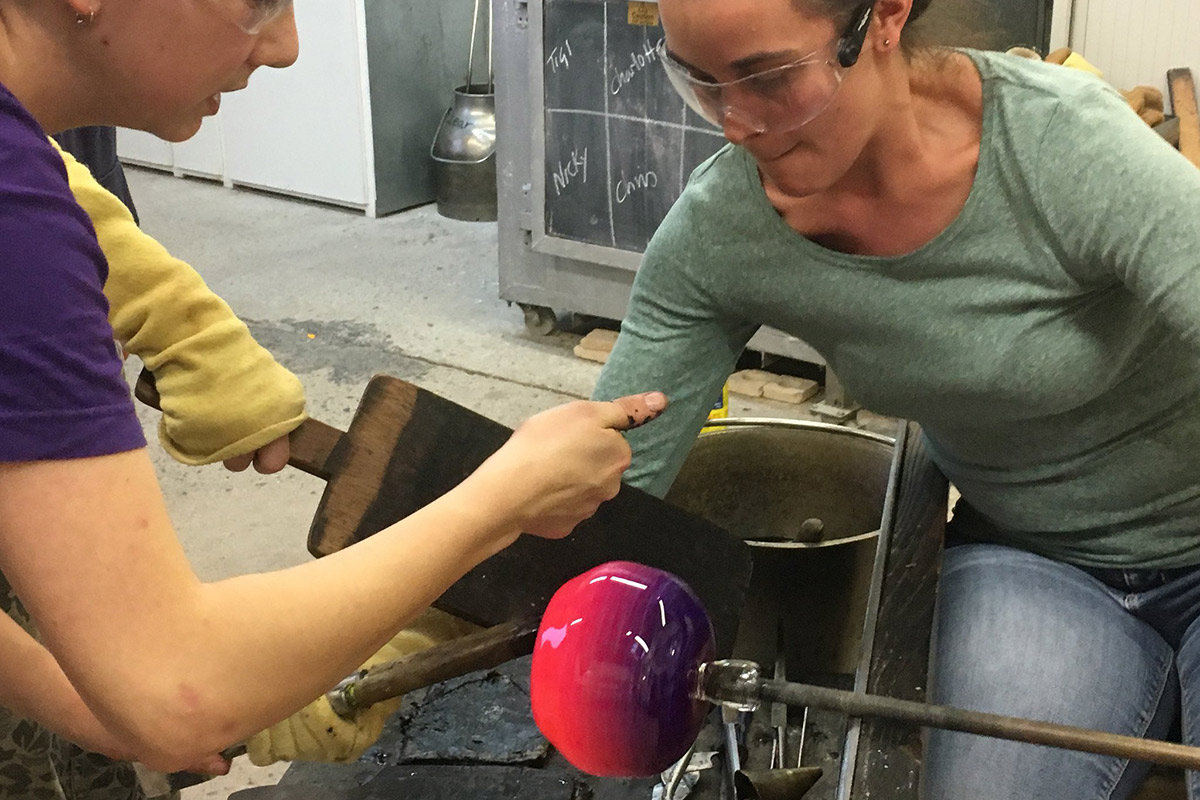This photograph captures a detailed moment of three individuals engaged in the intricate art of glassblowing. Central to the image is a glowing piece of molten glass attached to a rod, transitioning in color from dark bluish-purple on the right to pink on the left. One woman, prominently featured leaning towards the camera, wears clear safety goggles, a green long-sleeve shirt, and blue jeans. She is shaping the vivid glass formation with a tool over a cylindrical metal chamber. Her focused expression and stance suggest a meticulous and skilled approach.

To her right, a second participant in a purple shirt is also engaged in shaping the glass, using a tool to aid in the process. The third individual, partially visible on the far left, wears a yellow sleeve and has a black-stained hand holding a wooden paddle, contributing to the collaborative effort. This dynamic scene, where safety gear, detailed craftsmanship, and coordinated teamwork blend seamlessly, vividly illustrates the complex and beautiful process of glassblowing.